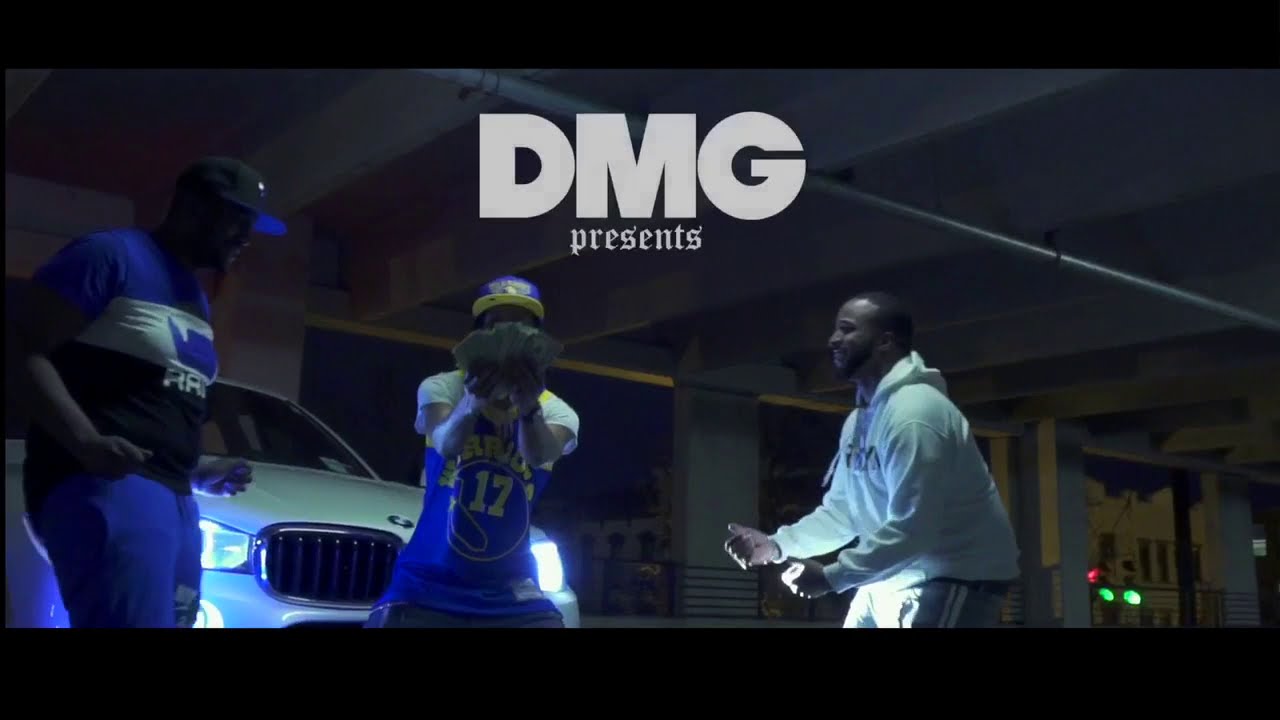This screenshot is likely from a rap music video or an advertisement. It features three African American men standing in a parking garage, with the nighttime sky visible in the background. The top of the image prominently displays in bold, white capital letters "DMG Presents." 

The man in the middle is dressed in a blue Golden State Warriors basketball jersey with the number 17 and a matching blue and yellow baseball cap. He holds a fan of cash in his hands, partially covering his face. To his left, there's a man wearing a black baseball cap with blue trim, a blue, white, and black short-sleeved shirt, and blue pants. On the right, another man is dressed in a primarily white hoodie with gray sweatpants and appears to be smiling. They are positioned in front of a white BMW sedan with its headlights on, adding to the urban and stylish atmosphere of the shot.